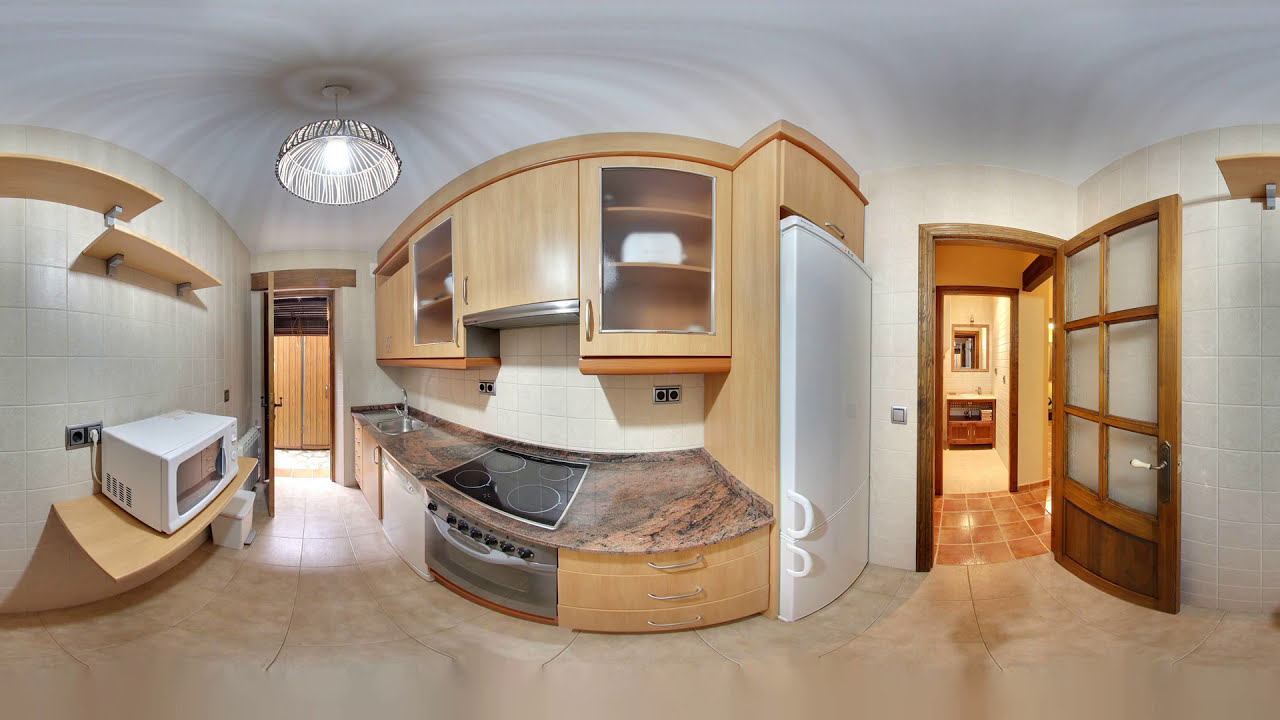This panoramic 360-degree image captures a spacious kitchen, offering an extensive view from left to right. At the far left, a white microwave oven sits on a pale wooden shelf mounted on a wall adorned with checkered white tiles. Above the microwave, two additional shelves are fixed to the tiled wall. The floor beneath is a beige tile that complements the walls. Moving towards the middle, there's an open door leading to an adjacent room; a ceiling light fixture illuminates this area. Centrally, a countertop and light wood cabinetry house a stovetop and an oven, accompanied by glass shelves above and more wooden shelves flanking the oven. A white dishwasher is also present among the appliances. Continuing to the right, a white refrigerator is placed with its handles towards the bottom of the image, next to another doorway framed with darker wood. This door opens into another room where the floor tiles shift to a darker brown and a cabinet area with a mirror can be seen. Additional cabinetry and another open door are visible towards the far right, completing the panoramic view with a continuation of the white tiled walls and the white ceiling that showcases swirly shadow patterns created by the light fixture.